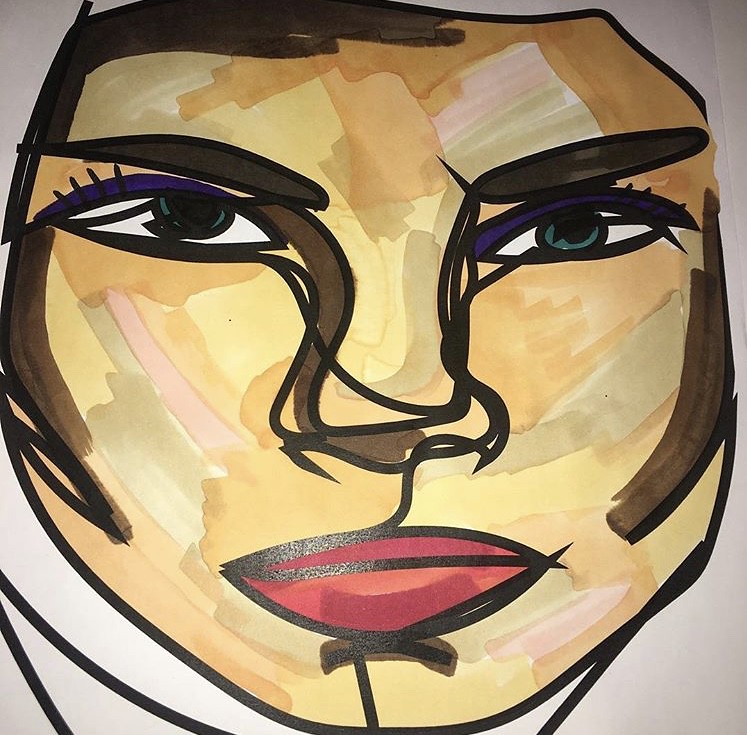This is a stylized drawing of a woman's face created using marker pens. The woman appears to be wearing either a headscarf or hoodie, indicated by the gray outline surrounding her face. Her facial features are prominently outlined in black, capturing a striking and bold visual effect. 

Her eyebrows are dark brown and well-defined, contrasting with her vivid green eyes. The artist has used several loose lines to shape her nose, seamlessly merging into the lines that define her mouth. She has a full lower lip and a thinner upper lip, with additional lines suggesting the contour of her chin. 

The woman's brown hair subtly peeks into the composition at both the left and right edges. Her skin is a complex mix of multiple colors, including shades of orange, yellow, pink, white, and beige, which together provide a rich depth and texture to her visage.